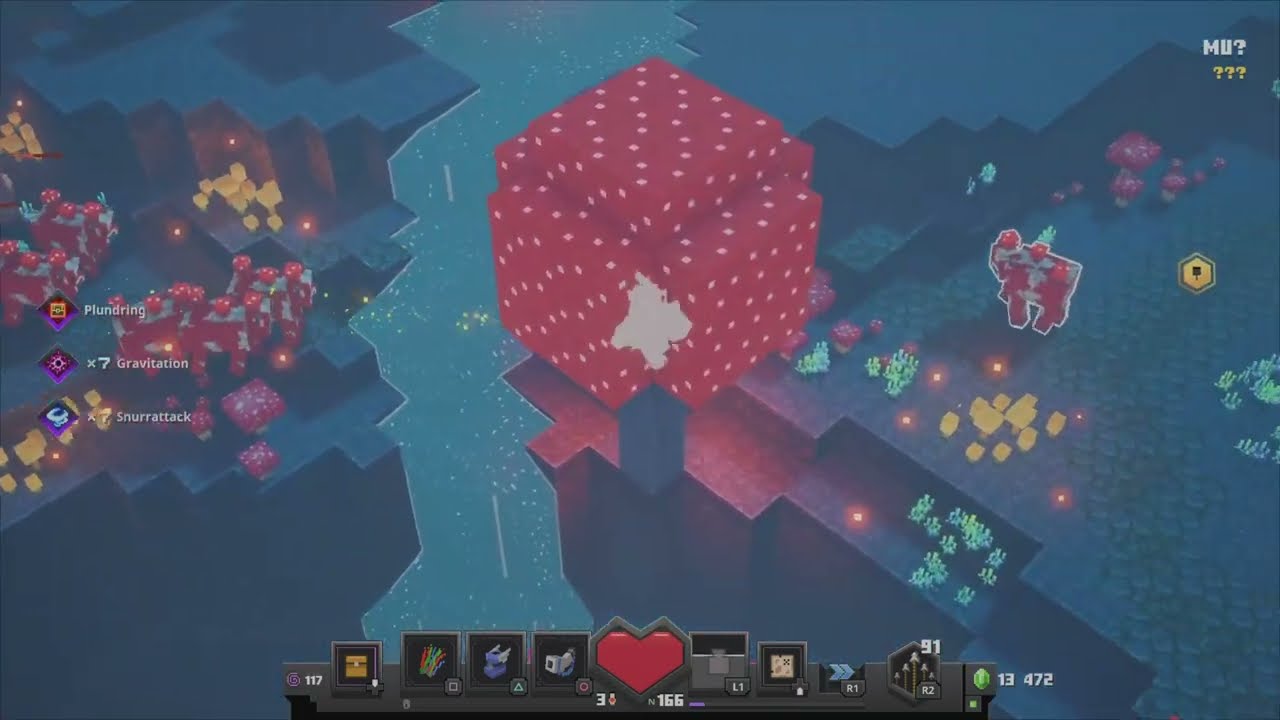The image is a vibrant screenshot from a video game, capturing a highly detailed and colorful scene. Dominating the center is a large red cube dotted with pink spots, resembling a strawberry. Smaller red objects are scattered around it, amidst yellow, green, and red shrubbery-like plants. The background features terraced geometric shapes with slate-gray and light-blue elements, possibly depicting a river splitting the scene slightly left of center. Below the red cube, a series of multicolored game-related emblems, including a purple, gold, red, blue, and green emblem, along with a distinct red heart shape, can be seen. The top right corner of the screen displays text reading “MU?” followed by three smaller question marks. On the left side of the screen, there is a notification or control panel listing "plundering," "gravitation," and "snare attack," adding to the immersive and interactive feel of the game environment.